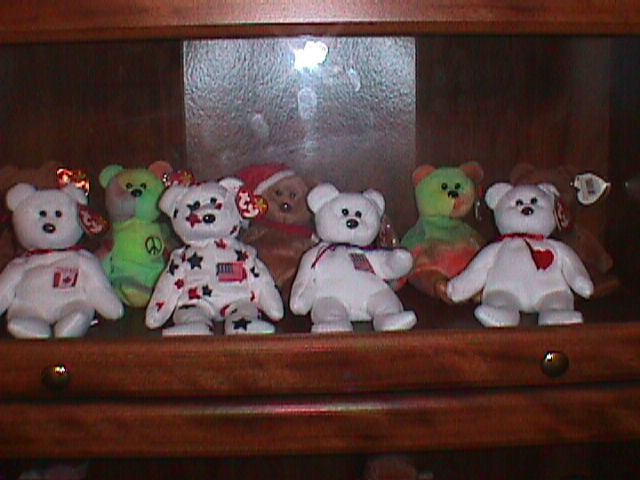In this photograph, a collection of Beanie Baby bears is meticulously arranged on a wooden shelf enclosed in a mahogany display case with a glass front, featuring two small handles for opening. The front row showcases four white Beanie Babies: one adorned with a Canadian flag on its chest, another decorated with red and blue stars alongside the American flag, a third with an indistinguishable flag, and a fourth featuring a simple red heart. Behind them are five more Beanie Babies, comprised of three brown and two tie-dye bears. The brown bears include a fuzzy one, another wearing a Santa hat with a red scarf, and a plain one, while the tie-dye bears vary with one being green and pink, and the other in green, yellow, and purple hues marked by a peace sign. With their iconic Ty heart tags still attached to their ears, these miniature bears, all sporting black eyes, appear to form a cherished collection.